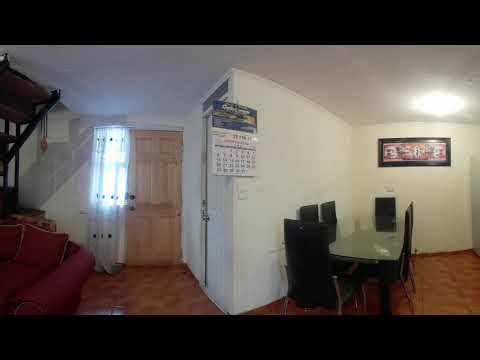The photograph captures a wide-angle shot of the interior of a home, showcasing both the living room and dining room areas. To the left, a red couch is partially visible near a light wood-colored door, likely the front entrance, accompanied by a small window. Adjacent to this is another door, probably leading to a bedroom. Behind the couch, the walls and ceiling are white, extending a sense of space and brightness. In the center, a calendar is noticeable on the wall, marking the transition between the two rooms.

On the right side, the dining area features a glass-top table surrounded by six black chairs. Above the table, a long rectangular photograph or painting in a black frame is prominently displayed under a bright yellow ceiling light. The rich wood-colored or laminate flooring throughout the space contrasts the lighter shade of the door, adding warmth and coherence to the scene.